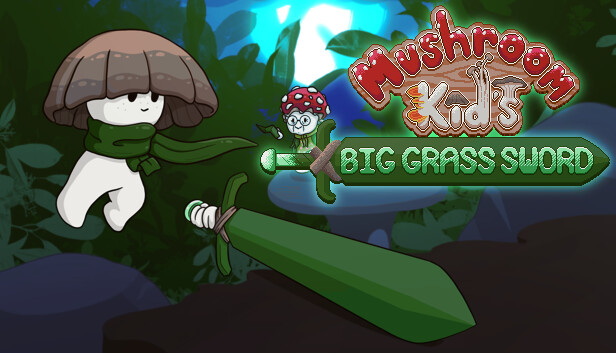The image depicts a cartoon or anime-style scene, possibly from a video game or children's cartoon, featuring anthropomorphic mushrooms. Dominating the left side is a character designed as a white-bodied mushroom with a dark brown mushroom cap as a hat, and a distinctive green scarf tied around its neck. The mushroom character has two black circular eyes and stands on two legs. Extending from its right side, it wields a large green sword with a white-wrapped handle. In the middle right, another sword, also green, has a sign affixed to it that reads "BIG GRASS SWORD" in light green capital letters. Above this, a prominent logo reads "Mushroom Kids." The word "Mushroom" appears in a stylized red, puffy, cloud-like font adorned with white dots, while "Kids" is white with mushroom details integrated into the letters. Additionally, there is a small mushroom character with a red cap and white dots, wearing glasses, situated somewhere in the background. The overall scene suggests a whimsical and imaginative setting, likely aimed at a younger audience.